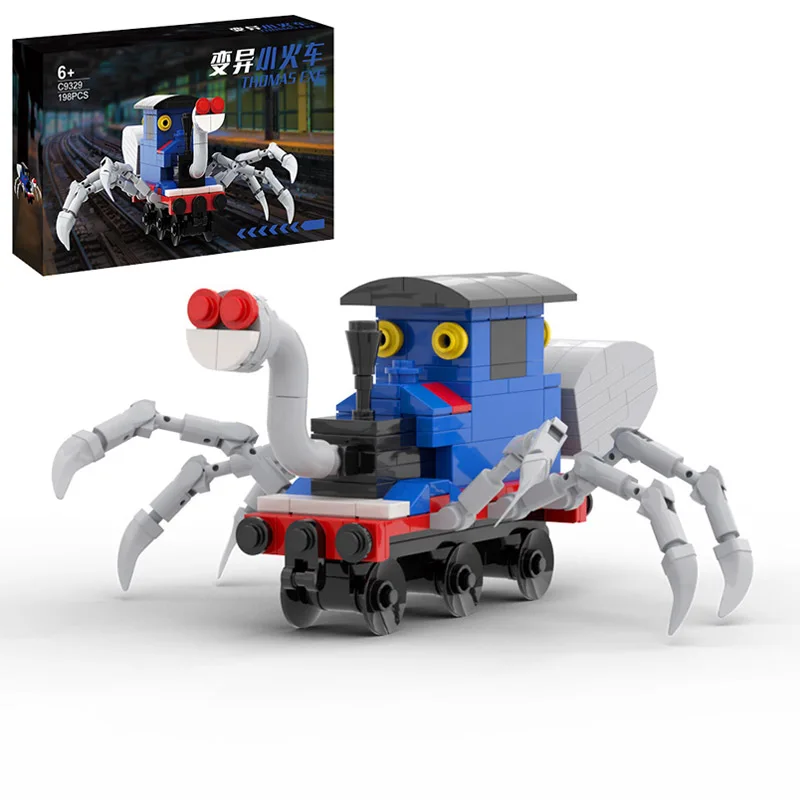In the image, we see a detailed and colorful children's construction model inspired by Thomas the Tank Engine. The model is reminiscent of a Lego set but seems to be from a distinct foreign brand, possibly Asian, with a name that could be interpreted as "Thoomas EXE." It appears to be an advanced toy, designed for children aged six and up, comprising 195 pieces.

The train-like model features a vibrant blue body with a red base, complemented by black wheels and gray hubs. The front of the train is adorned with three black knobs mimicking lights, and the smokestack is a striking gray. Unique to this model, it has six articulated white arms, three on each side, akin to crab legs. These add a playful, creature-like quality to the design.

Further adding to the whimsy, the front of the train sports a red-colored snout with an insect-like white "butt" at the rear. It has yellow eyes set in a black roof, giving it an anthropomorphic appearance. The model also includes a black cube located near the head of the train, adding to its intricate details.

The background of the image is minimal, with only a shadow cast by the train model on the platform, emphasizing the toy itself. In the top left corner, the box of the model can be seen, featuring an image of the assembled toy along with various texts, including some in Asian characters, possibly Chinese or Japanese. The bottom left of the box indicates the number of pieces and other relevant information, framing the detailed and imaginative design of this unique toy model.